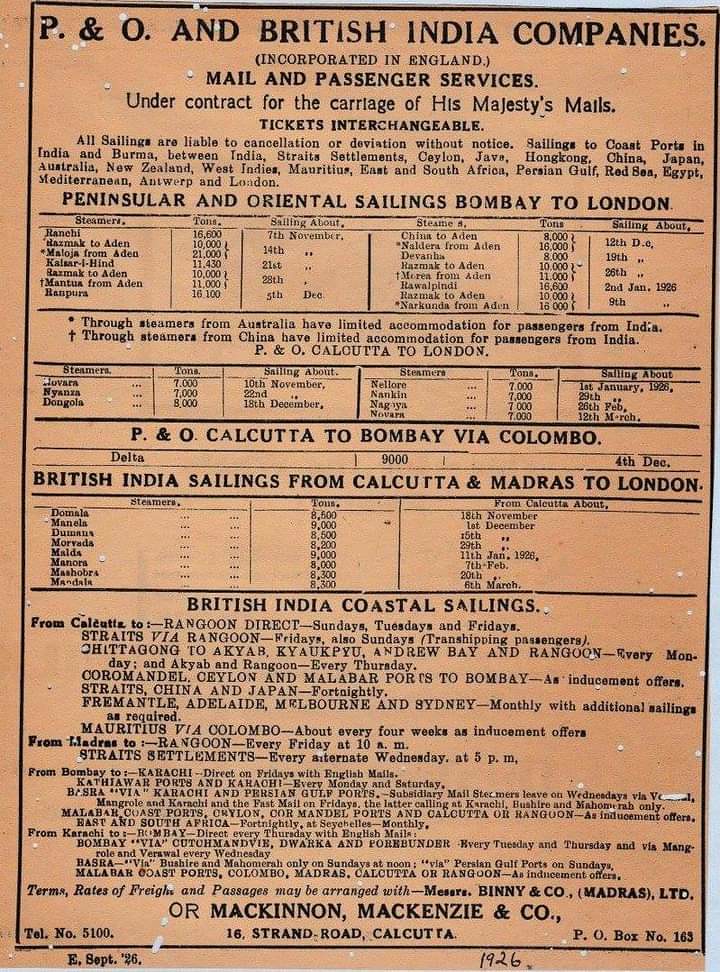The image is a scan or photograph of a document on a reddish-orange background, detailing various maritime services. At the top, in large black capitalized text, it reads "P&O and British India Companies." Beneath that, it states "Incorporated in England" followed by "Mail and Passenger Services." It further mentions, "Under contract for the carriage of His Majesty's mails." The document specifies, "Tickets Interchangeable" and includes a caveat, "All sailings are liable to cancellation or deviation without notice." There is a comprehensive list of destinations, including "Sailings to coast ports in India and Burma, between India, Straits, Settlements, Keilung, Java, Hong Kong, China, Japan, Australia, New Zealand, West Indies, Mauritius, East and South Africa, Persian Gulf, Red Sea, Egypt, Mediterranean, Antwerp and London."

Immediately below, in large black text, is the header "Peninsular and Oriental Sailings, Bombay to London." Below this, three organized charts outline various routes and schedules. The first chart under the heading "P&O, Calcutta to Bombay via Colombo" details a single date and time. The second chart, labeled "British India Sailings from Calcutta and Madras to London," lists multiple places, times, and dates. The last section provides information on "British India Coastal Sailings," but the text is too small to read. At the very bottom of the document are the details "OR, McKinnon, McKenzie, and Co." followed by the address "16 Strand Road, Calcutta."